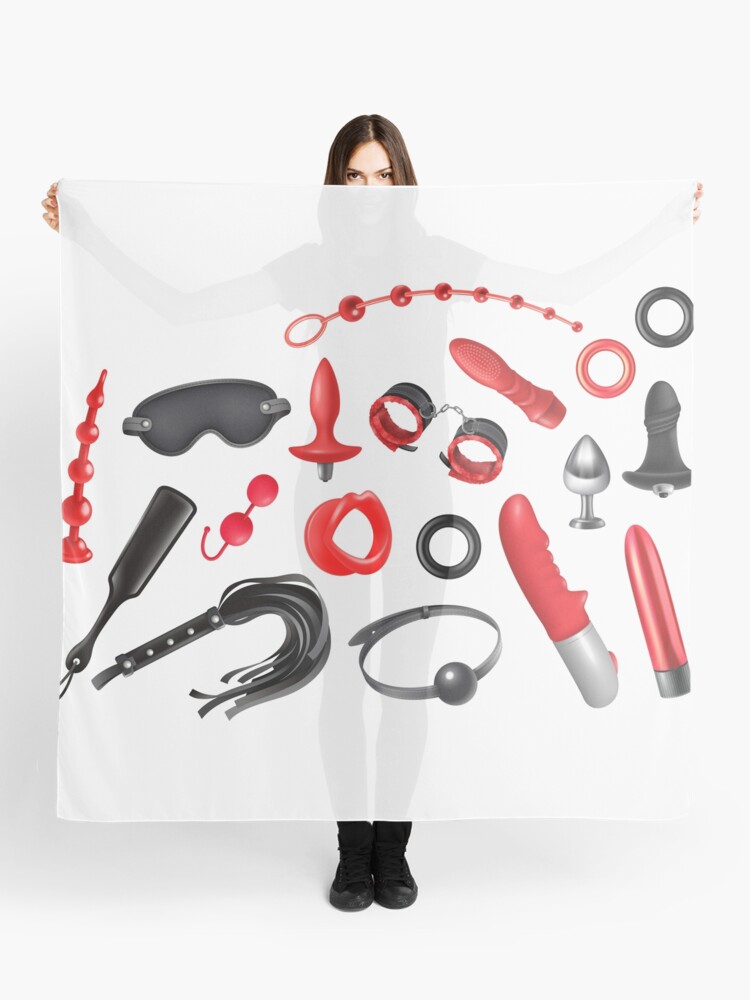The image is a color photograph featuring a woman with long brown hair standing in front of a plain white background. She is holding up a large, transparent fabric tapestry that drapes from her extended arms, obscuring her body while allowing her silhouette to be faintly visible through the material. The tapestry is adorned with an array of explicit sexual objects mainly in black and red, including a face mask, a choke collar with a ball gag, handcuffs, ball and chains, whips, and various dildos. Her serious expression is partially visible, showing her eyes and upper face, while she wears dark shoes. The detailed collection of items on the fabric suggests they are tools associated with BDSM activities, adding a provocative element to the otherwise minimalistic composition of the image.